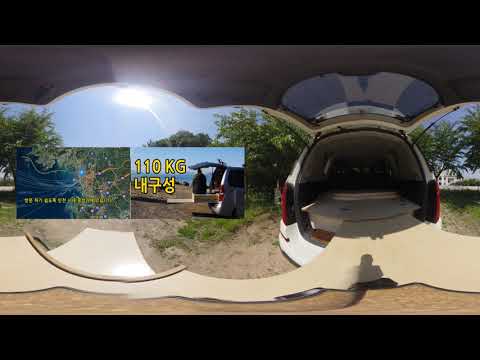The image shows a white SUV with its trunk open and some of the seats folded down, likely in preparation for loading items. The SUV's interior is beige. The scene is set outdoors on a dirt terrain surrounded by various foliage and trees, under a bright blue sky with sunlight beaming from the left side. There is a shadow of a person visible at the bottom of the photograph. The image has some lens artifacts or distortion, and features thin black bars at the top and bottom. An overlay on the right side of the image displays "110 KG" in yellow text with a black outline, followed by text in characters resembling Chinese or Japanese. Additionally, a small thumbnail on the middle left shows an aerial view of a map.